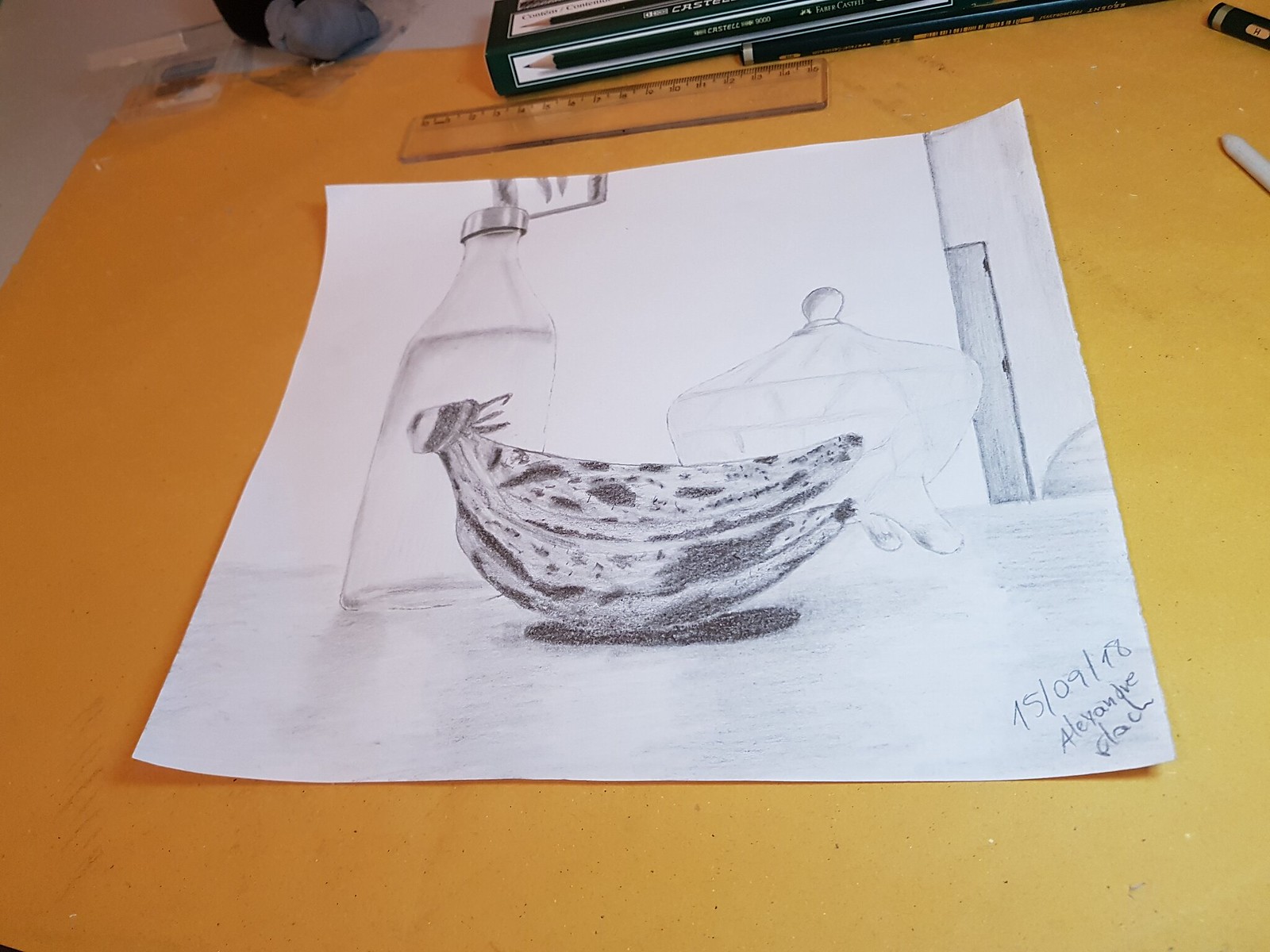This pencil sketch, masterfully crafted, showcases a variety of objects arranged on the surface of a table, each element rendered with intricate detail. The focal point of the artwork is a bunch of ripe bananas, beautifully drawn with realistic shadows cast beneath them. In the background, a bottle filled with liquid, likely water, adds depth to the composition. Nearby sits a sugar bowl, distinguished by its decorative edges and lid. The scene extends to the corner of a room, marked by a door with visible hinges, and a wall adorned with a picture. Every object, including the table surface, is meticulously shaded to enhance the realism. Notably, the piece is dated "1509-18" and signed "Alexander," though the artist's signature, appearing as "D-A-C-H," is uniquely stylized and somewhat difficult to decipher. The sketch itself is displayed on a blotter, surrounded by additional drawing tools such as a ruler and various pens and pencils, further adding to the setting's authenticity.